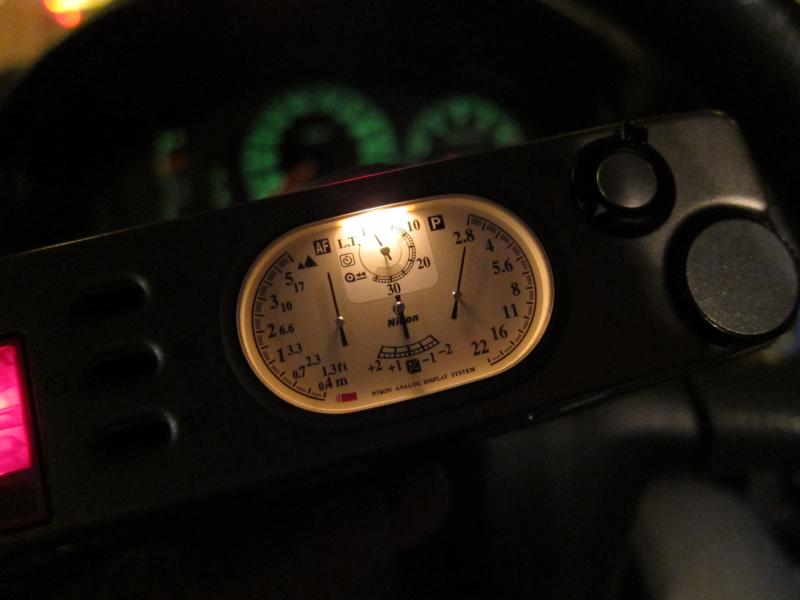This image showcases a close-up view of a Nikon analog display system, prominently featuring a dial with black numeric markings and indicator hands. In the center, "Nikon" is clearly inscribed, confirming the brand. One hand on the left side points to "AF," which stands for Auto Focus, while the opposing hand on the right side is directed at the number "2.8." The dial also includes a series of aperture values arrayed in a semi-circle: 4, 5.6, 8, 11, 16, and 22. Additionally, the bottom of the dial displays the text "analog display system." On the left side of the dial, another set of numerical values corresponds to various distances and focal lengths, including 5, 17, 3, 10, 2, 6.6, 1, 3.3, 0.7, 2.3, and 1.3 feet, with a final metric measurement of 0.4 meters. This detailed view emphasizes the precision and variety of settings available on the Nikon device.